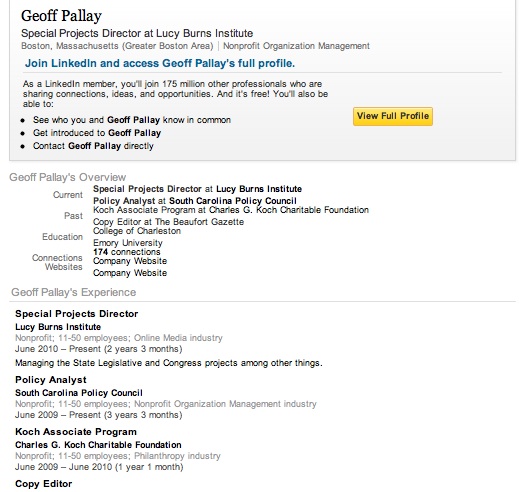This image portrays a LinkedIn profile preview for Jeff Pallay. The page features a clean, white background with a gray header box at the top. The header area presents Jeff Pallay's name in bold black text, with a phonetic spelling provided as "G-E-O-F-F-P-A-L-L-A-Y." His title is also listed: Special Projects Director at the Lucy Burns Institute, located in the Greater Boston Area, specializing in Nonprofit Organization Management.

A prominent call-to-action in blue invites viewers to join LinkedIn to access Jeff Pallay's full profile. It notes that, as a LinkedIn member, you will join 175 million other professionals sharing connections, ideas, and opportunities—for free. Additional features include the ability to see shared connections with Jeff Pallay, get introduced, and contact him directly, highlighted by a yellow "View Full Profile" button.

Below the header, the profile overview includes details of Jeff Pallay's current roles: Special Projects Director at the Lucy Burns Institute, policy analyst at the South Carolina Policy Council, a Kosh Associate Program member at the Charles G. Kosh Charitable Foundation, and a copy editor position at the Beaumont Gazette. His educational background is listed, including institutions like the College of Charleston and Emory University. He has 174 connections, and the profile also mentions links to a company website.

Jeff Pallay's professional experience is outlined with specific roles and durations:
- Special Projects Director at the Lucy Burns Institute (June 2010 to present, two years and three months), where he manages the State Legislative and Congress Projects among other responsibilities.
- Policy Analyst at the South Carolina Policy Council (June 2009 to present, three years and three months).
- Kosh Associate Program participant (June 2009 to June 2010).